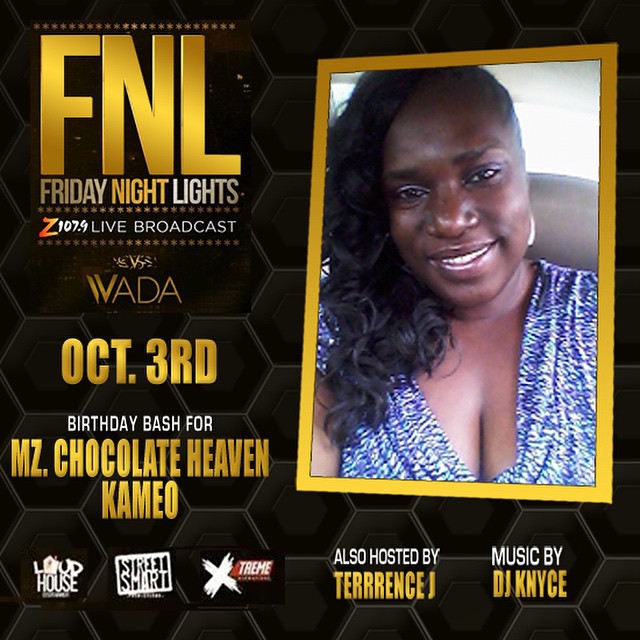The image is a vibrant advertisement for a birthday party event, set against a striking black background featuring a hexagon pattern. Dominating the right side of the image is a large photo of an African American woman, presumably the birthday girl, wearing a blue shimmering dress. Her hair is styled to one side, and she smiles warmly at the camera, adding a personal and joyful touch to the scene. In the top left corner, the bold, golden text "FNL" stands out, accompanied by "Friday Night Lights" and "Z107.9 Live Broadcast vs WADA." Below these details, the date "October 3rd" is prominently displayed, marking the special event: a birthday bash for "MZ Chocolate Heaven Cameo." At the bottom left, logos for Loud House, Street Smart, and Xtreme add to the event's branding, while the bottom right reveals the names of the host, Terence J, and the DJ, DJ Nice. The overall design, with its luxurious gold lettering and thematic imagery, suggests a glamorous and exciting night to come.